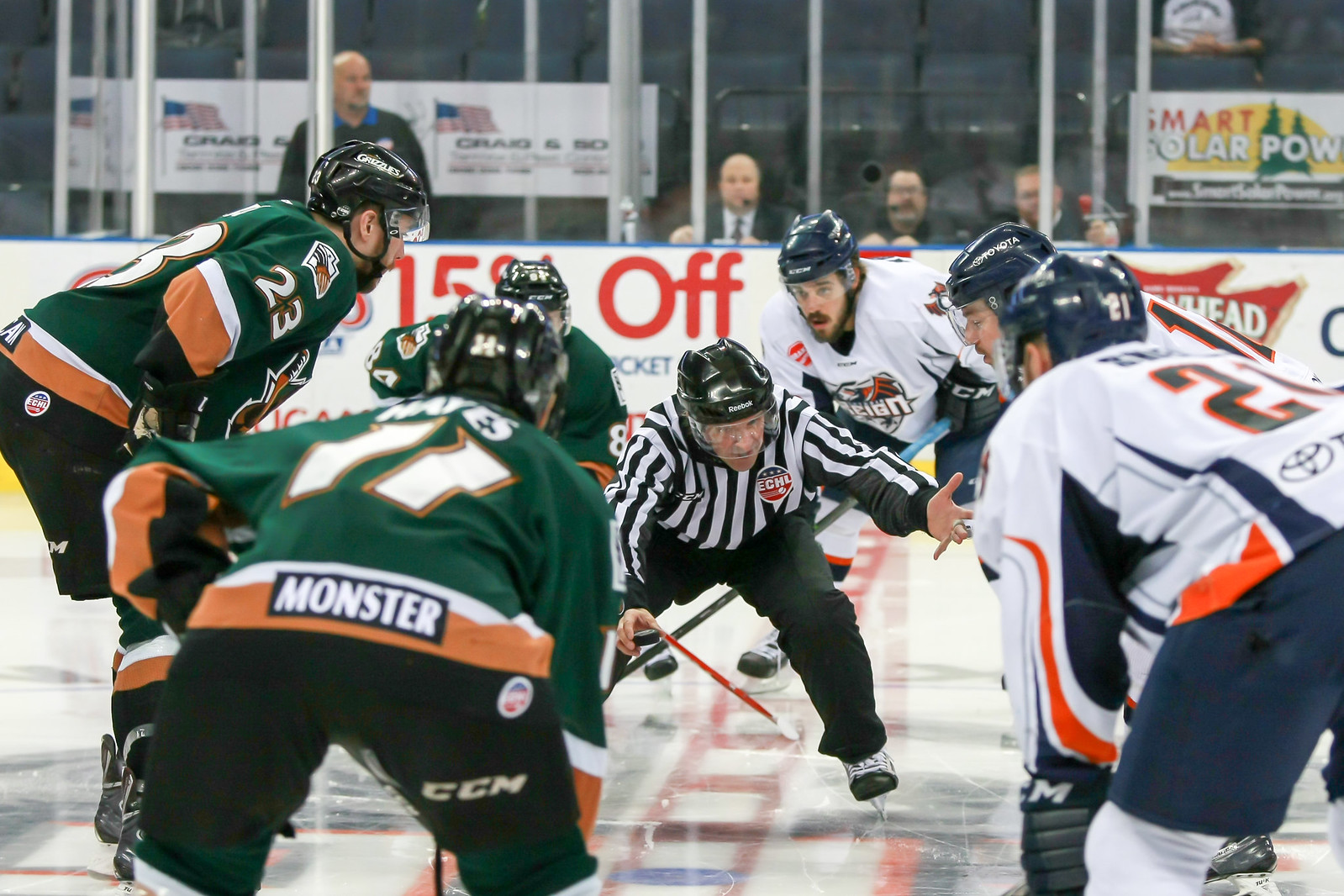The image captures an intense moment at an ice hockey game, focused on the referee poised at center ice about to drop the puck. Clad in a black and white striped shirt, black pants, a helmet, and skates, the ref stands surrounded by two competing teams. The team to his left is donned in green jerseys with brown bottoms, accompanied by black pants and helmets, while the team on the right showcases white jerseys with navy-colored shorts and helmets, accented with orange and blue stripes. The players are hunched over, eyes glued to the puck about to hit the ice, positioned on a distinctive red center line. In the background, a boundary wall adorned with advertisements and signs, including one featuring an American flag and the name "Craig," provides a backdrop to the scene. Above this wall, a plexiglass partition separates the rink from the spectators. Some watchers are visible—one standing and three seated—alongside a variety of signs, including an ad with a picture of a sun and trees, labeled "Smart Solar Power." The announcers are also visible, seated with microphones, likely narrating the intense, unfolding action on the ice.